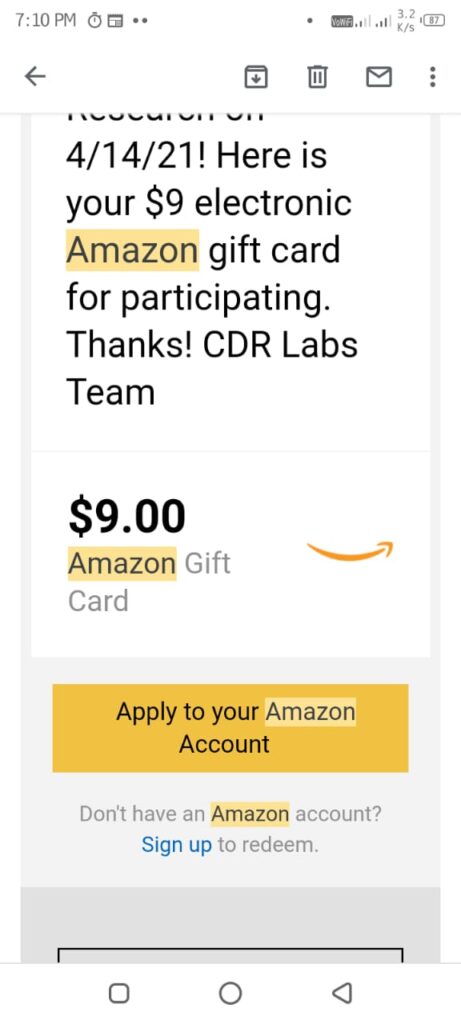At the top of the image, there is a status bar displaying various icons and information. On the left, there is a black arrow pointing to the left, followed by a black-outlined box with a white center and a downward-pointing black arrow, a black delete garbage can icon, an envelope outlined in black, and three vertical dots. In the center of the status bar, it shows the time as 7:10 p.m., accompanied by a small clock icon. To the right, there is a small black box indicating "Wi-Fi," with two signals colored in and three signals filled, and next to it, the display reads "3.2." There is also an outlined battery icon showing an 87% charge.

Below the status bar, an advertisement from Amazon is partially visible. The heading appears cut off but is written in black letters. The ad contains a message dated "4-14-21" with "here is your $9 electronic Amazon gift card for participating, thanks!” signed by the CDR Labs team. The word "Amazon" is highlighted in yellow throughout the message, while the rest of the text is in black on a white background.

The ad further breaks down the gift card value, stating "$9" in black letters, followed by "Amazon gift card," with "Amazon" highlighted in yellow. Below this, the familiar Amazon arrow logo is displayed in gold, curving upward against a white background with a gray shadow.

A gold banner beneath the gift card description bears the text "apply to your Amazon account" in black, with "Amazon" highlighted in a lighter yellow. Just below, there's a prompt: "don't have an Amazon account, sign up to redeem," where "Amazon" is again highlighted in yellow and "sign up" appears in blue, while the remaining text is gray.

At the very bottom of the image, there is a darker gray section with a black line at the bottom edge, where the navigation buttons for the back function are barely visible.